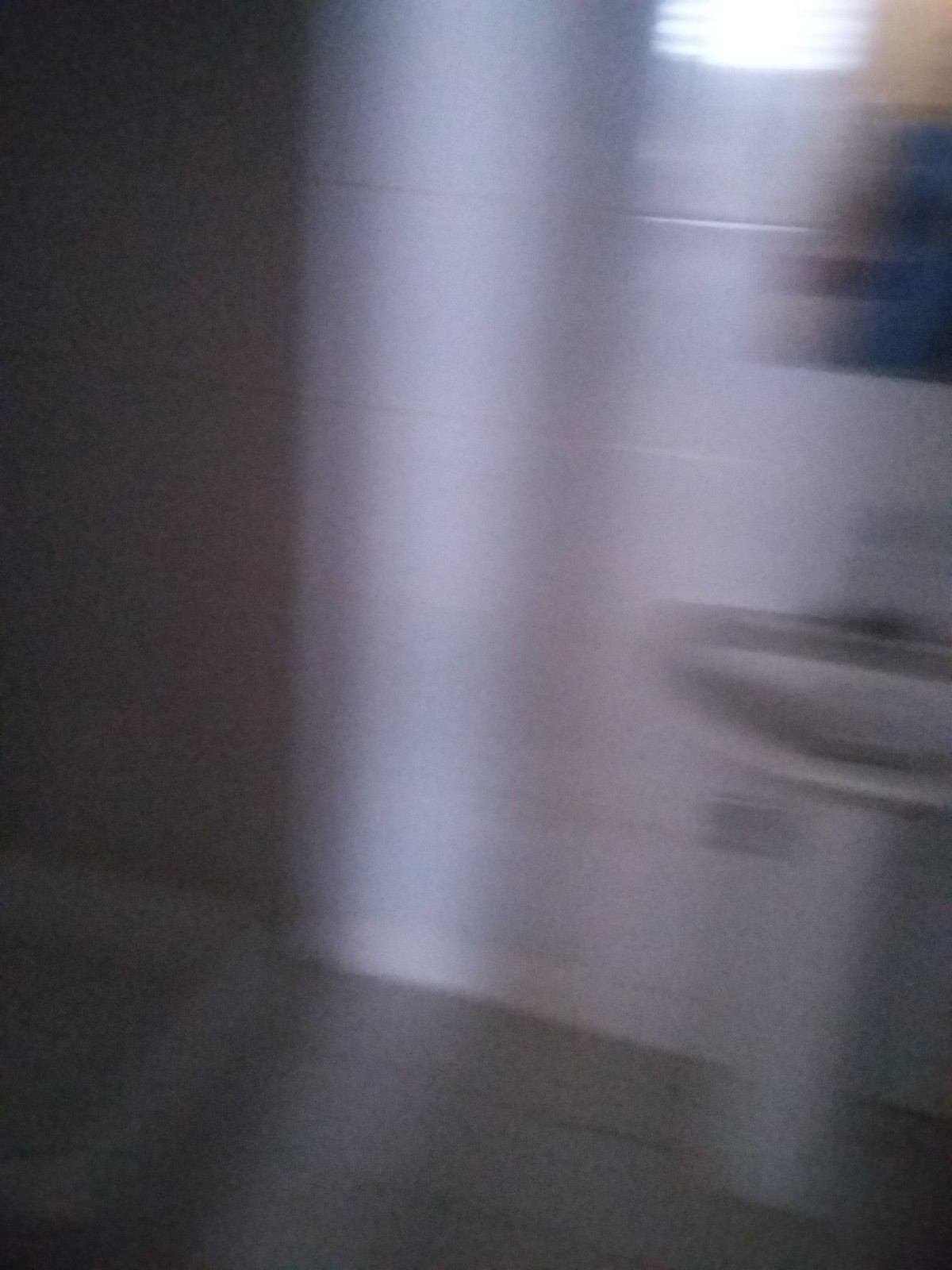A blurry, vertically oriented color photograph captures a scene that becomes discernible upon closer inspection. Positioned in the lower right quadrant of the image is a porcelain sink, standing against a white wall. The sink is bathed in soft highlights, particularly along the edges where the light meets the wall. Horizontal lines run across the wall, suggesting the presence of large bricks or tiles, indicative of a school bathroom setting. In the top right corner of the image, a window or light source illuminates the scene, bordered by a light brown color. The photograph has a slight magenta tint, and a blue object is vaguely visible in the upper right quadrant, adding to the enigmatic quality of the image.